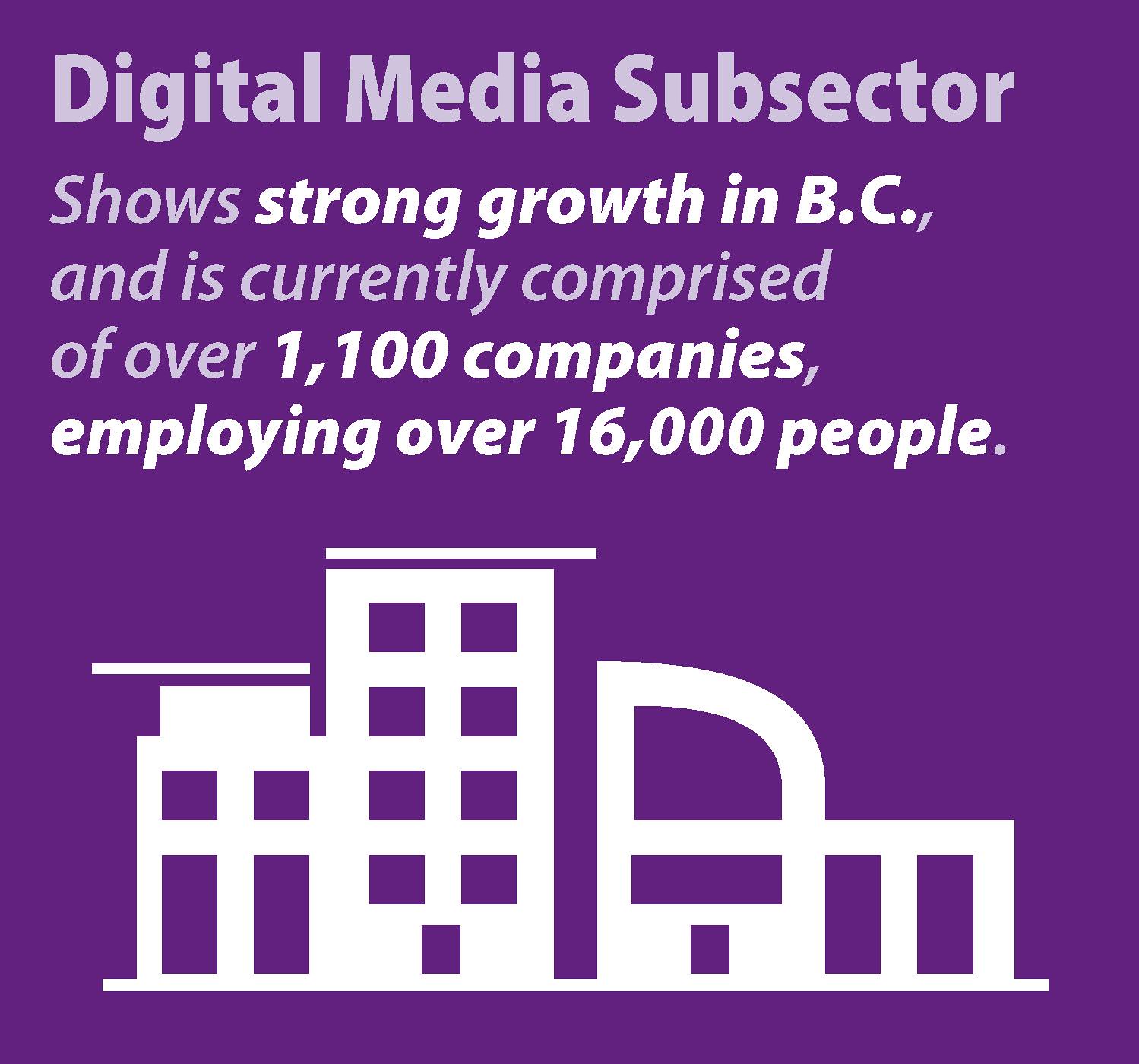The image features a predominantly purple background with text and graphic elements. At the top, in a grayish hue, the text reads "Digital Media Subsector." Below this, a detailed message is presented in alternating light purple and white fonts, stating: "Shows strong growth in BC and is currently comprised of over 1,100 companies employing over 16,000 people." The phrase "Shows strong growth in BC" and "employing over 16,000 people" are highlighted in white, emphasizing their importance. Beneath the text, there is a 2D silhouette of four white buildings, each outlined distinctly with purple windows, ranging from a small one-story structure on the far right to a taller four-story building near the center. One building to the center-right has a unique curved right edge, adding a touch of architectural variety. The stark white buildings against the purple background, with their uniform purple square and rectangular windows, provide a modern urban skyline representation, encapsulating the growth and dynamism of the digital media subsector in BC.